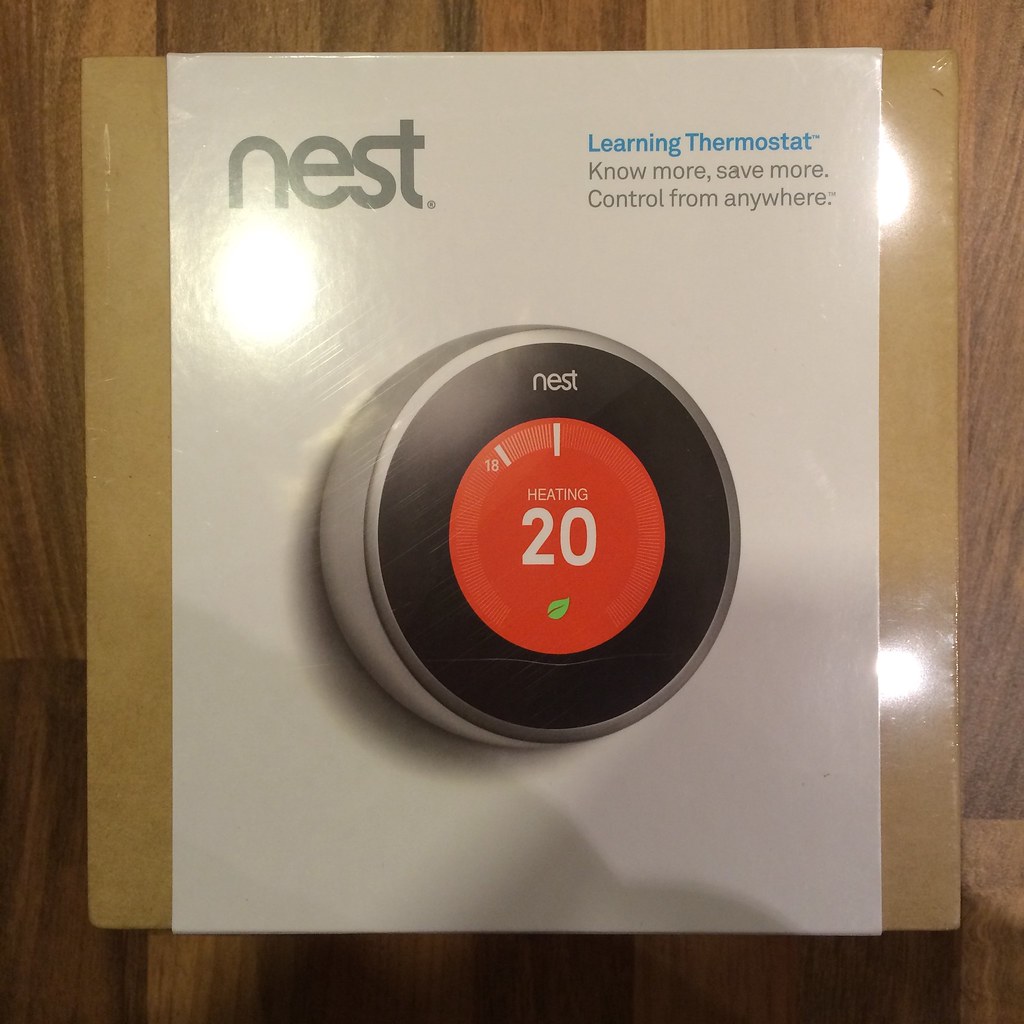In this image, we observe the packaging for a Nest Learning Thermostat displayed on a medium dark wooden surface, likely a table or countertop. The box, made of brown cardboard, prominently features a white label on the front. This label bears the text "Nest Learning Thermostat," along with key phrases like "No more, save more, control from anywhere." The label also includes an image of the thermostat itself, showcasing its sleek design. The device sports a silver housing and a black, all-digital face with no visible buttons, indicating that it is likely operated by rotating the outer ring. The display area of the thermostat is shown glowing red, presumably indicating the temperature or other relevant information. The prominently displayed "Nest" branding reinforces the product's identity.